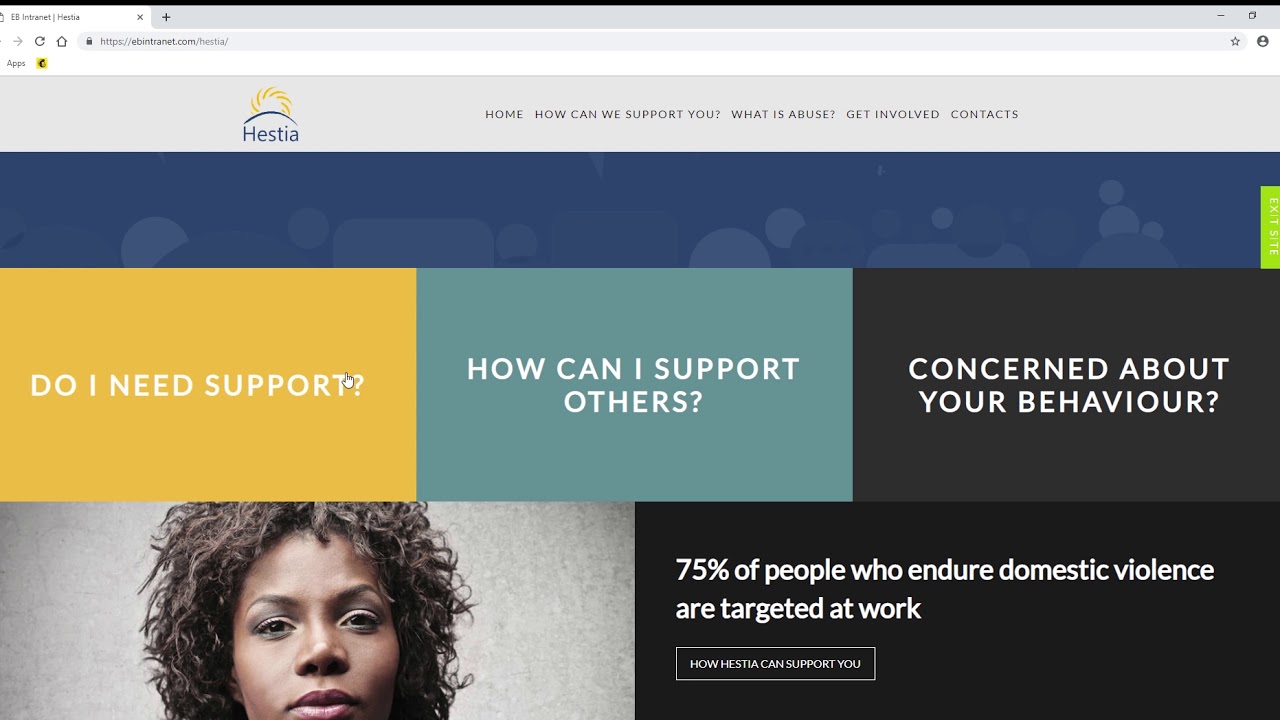The image appears to be a screenshot of a computer screen showcasing the homepage of a website named "Hestina," likely accessed through a specific intranet portal 'ebintranet.hestina'. At the uppermost part, the browser tab indicates the URL in partial text.

Below the browser tab, a gray navigation bar displays the website address "ebintranet.comHestina". Further down, the header features the Hestina logo, characterized by the text "Hestina" with a stylized, curved blue line and an icon resembling the sun above it. Adjacent to the logo, a navigation menu containing links titled "Home," "How Can We Support You," "What is Abuse," "Get Involved," and "Contact Us" is visible.

Beneath the header, a blue border adorned with circular shapes transitions to the main content area composed of three rectangular sections: 
1. A yellow rectangle titled "Do I Need Support?"
2. A light grayish-blue rectangle titled "How Can I Support Others?"
3. A black rectangle labeled "Concerned About Your Behavior?"

In the lower left corner of the image is a poignant photograph of an African American woman with dark, curly hair. She appears sorrowful, her expression reflective, and is set against a gray background.

To her right, a black rectangle exhibits a striking statistic: "75% of people who endure domestic violence are targeted at work". Further to the right, another rectangle invites users to explore "How Hestina Can Support You."